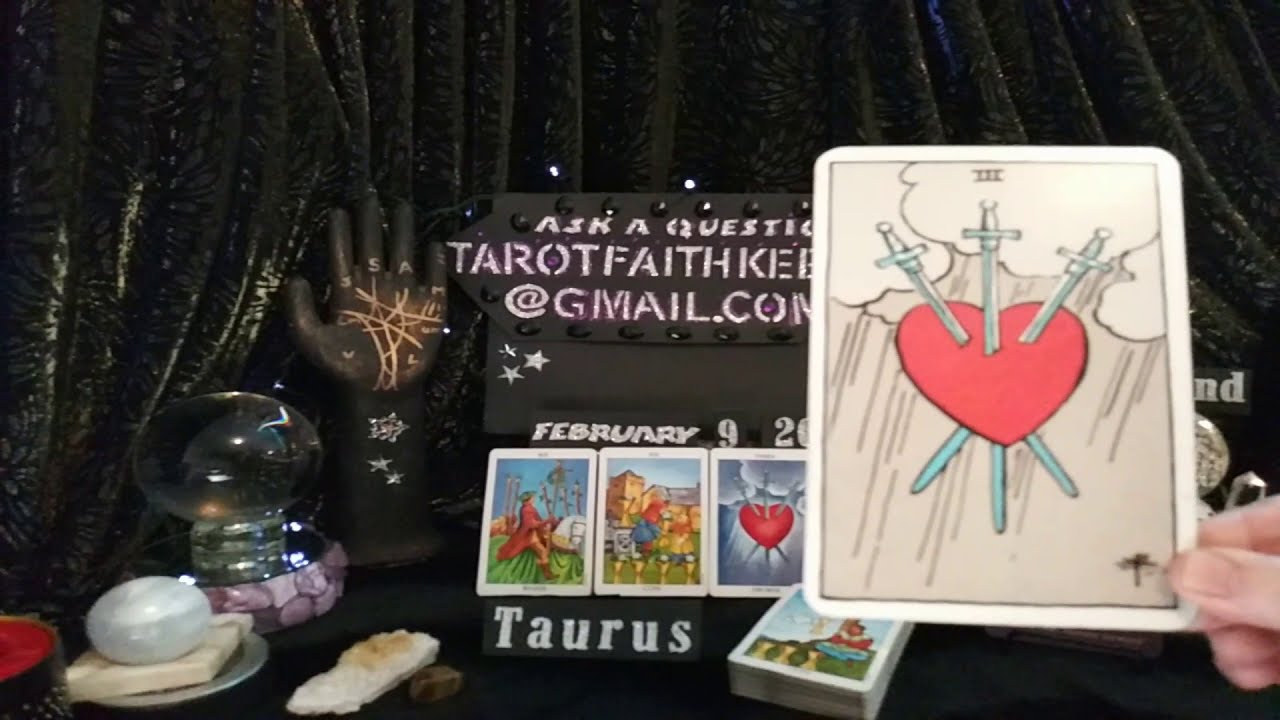In the image, a black curtain forms the backdrop, contrasting with a black table or surface in the foreground. Arranged on this table is an assortment of items reminiscent of a tarot reading setup. On the left-hand side, there's a small, round crystal ball, accompanied by other round objects. Behind these sits a pedestal hand statue, intricately designed with lettering and symbols on its palm and fingers. 

At the center of the display is a black plaque, prominently featuring the text "Ask a question," though the message is partially obscured. Following this, the email "tarotfaithkeb at gmail.com" can be seen but is also somewhat cut off. Below this, the word "Taurus" is displayed in white letters. There are three tarot cards beneath this text, each depicting a distinct image: one has a person, the middle one shows a building, and the third one—also held by a hand on the right side of the image—features a pink heart pierced by three swords, set against a backdrop of clouds and rain.

The setting appears stylized as an advertisement for tarot card readings, employing a varied color palette including black, white, gray, yellow, red, green, blue, purple, pink, and tan. The objects in the image are centrally positioned, creating a balanced composition.